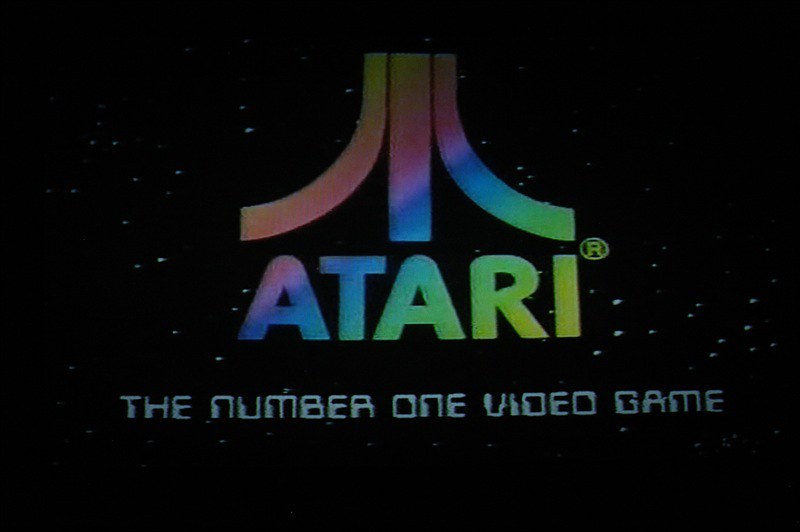The image depicts a predominantly black background, resembling a screen from a retro video game system or console. The dark backdrop is adorned with small, white specks, evocative of stars scattered across a night sky. Centrally positioned is a prominent rectangular shape flanked by two symmetrical shapes that begin as rectangles but curve outwardly away from the central form.

These shapes exhibit a shared gradient color pattern. Starting at the top, hues transition from greenish or light yellow, then gradually move into shades of brown, red, and purple, before blending into blues and greens towards the bottom. Below the central rectangular shape, the word "Atari" is prominently displayed in capital letters, adorned with the same gradient color pattern featured above. Beneath "Atari," in stark white capital letters, is the phrase "THE NUMBER ONE VIDEO GAME." Positioned to the right of the "I" in "Atari," there is a small circle containing the letter "R," indicating a registered trademark.